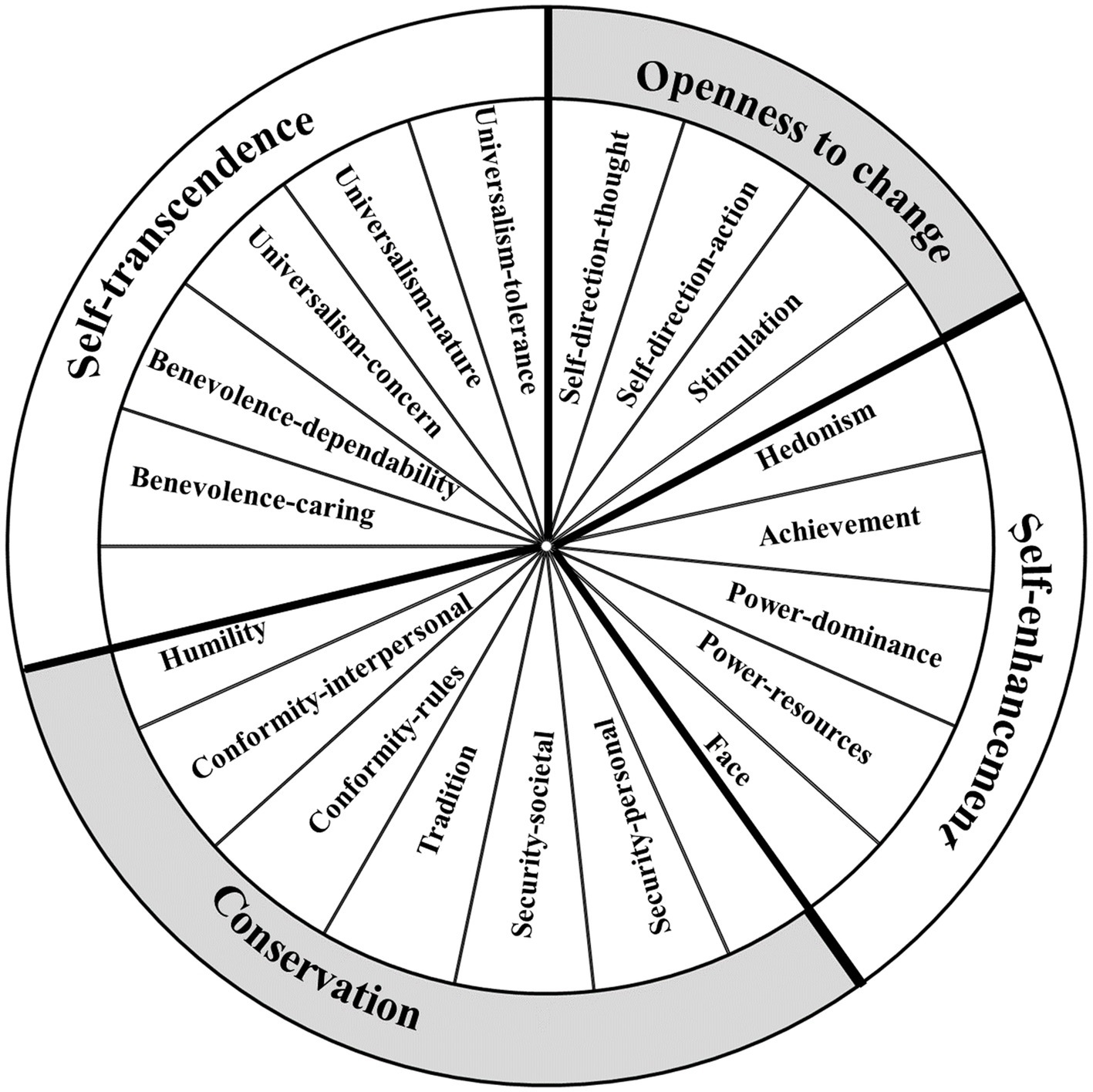The image features a large gray wheel segmented into multiple sections with black lines and text on a white background. This wheel is framed by four broader labels on its outer edge: "Openness to Change" in the top right, "Self-Enhancement" in the bottom right, "Conservation" in the bottom left, and "Self-Transcendence" in the top left. Each of these categories further subdivides into specific values arranged in a clockwise manner starting from the top left. Within "Openness to Change," we find "Self-Direction Thought," "Self-Direction Action," and "Stimulation." The "Self-Enhancement" sector includes "Hedonism," "Achievement," "Power-Dominance," "Power-Resources," and "Face." "Conservation" encompasses "Humility," "Conformity-Interpersonal," "Conformity-Rules," "Tradition," "Security-Societal," and "Security-Personal." Lastly, in the "Self-Transcendence" section, the values are "Universalism-Concern," "Universalism-Nature," "Universalism-Tolerance," "Benevolence-Caring," and "Benevolence-Dependability." The structured wheel appears to illustrate a taxonomy of values, possibly related to a research study.